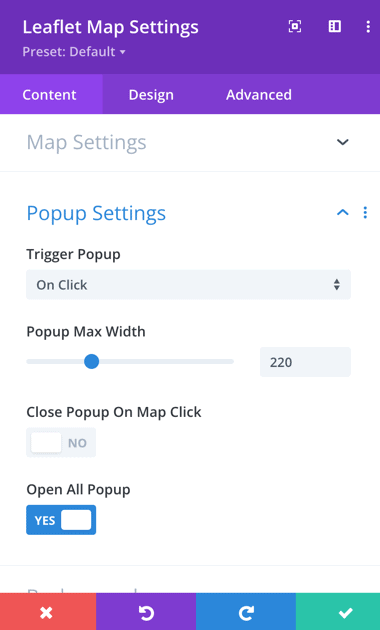This image appears to be a screenshot taken on a smartphone, showcasing the interface of a mobile application related to map settings. At the top of the screenshot, there's a purple header that indicates the application is handling "Leaflet Map Settings". The header features several tabs, including "Content", "Design", and "Advance", which seem to be sections that provide various options for customization. The "Content" tab is currently selected.

Below the header, the user can select different settings, such as "Map Settings" and "Pop-up Settings". The "Pop-up Settings" section is active, with several sub-options displayed:

1. **Trigger Pop-up**: This appears to be an option that can be toggled on or off.
2. **Pop-up Max Width**: This setting is configured to a value of 220.
3. **Close Pop-up on Map Click**: This option also seems to be toggleable, likely providing a choice between enabling or disabling it.
4. **Open All Pop-ups**: The option to enable this is indicated, but there are no visible checkmarks or indicators for whether it is active or not.

At the bottom of the interface, there is a row of icons featuring an "X" in red and purple, which might be used to close the settings or cancel changes, a blue arrow pointing to the right, likely for navigation or advancing to the next screen, and a green checkmark which may be for confirming changes or saving the settings.

Overall, the screenshot demonstrates various configuration options available for customizing map interactions and pop-ups within this specific application, although the exact purpose and functionality of the "Leaflet Map Settings" are not entirely clear based on the image alone.